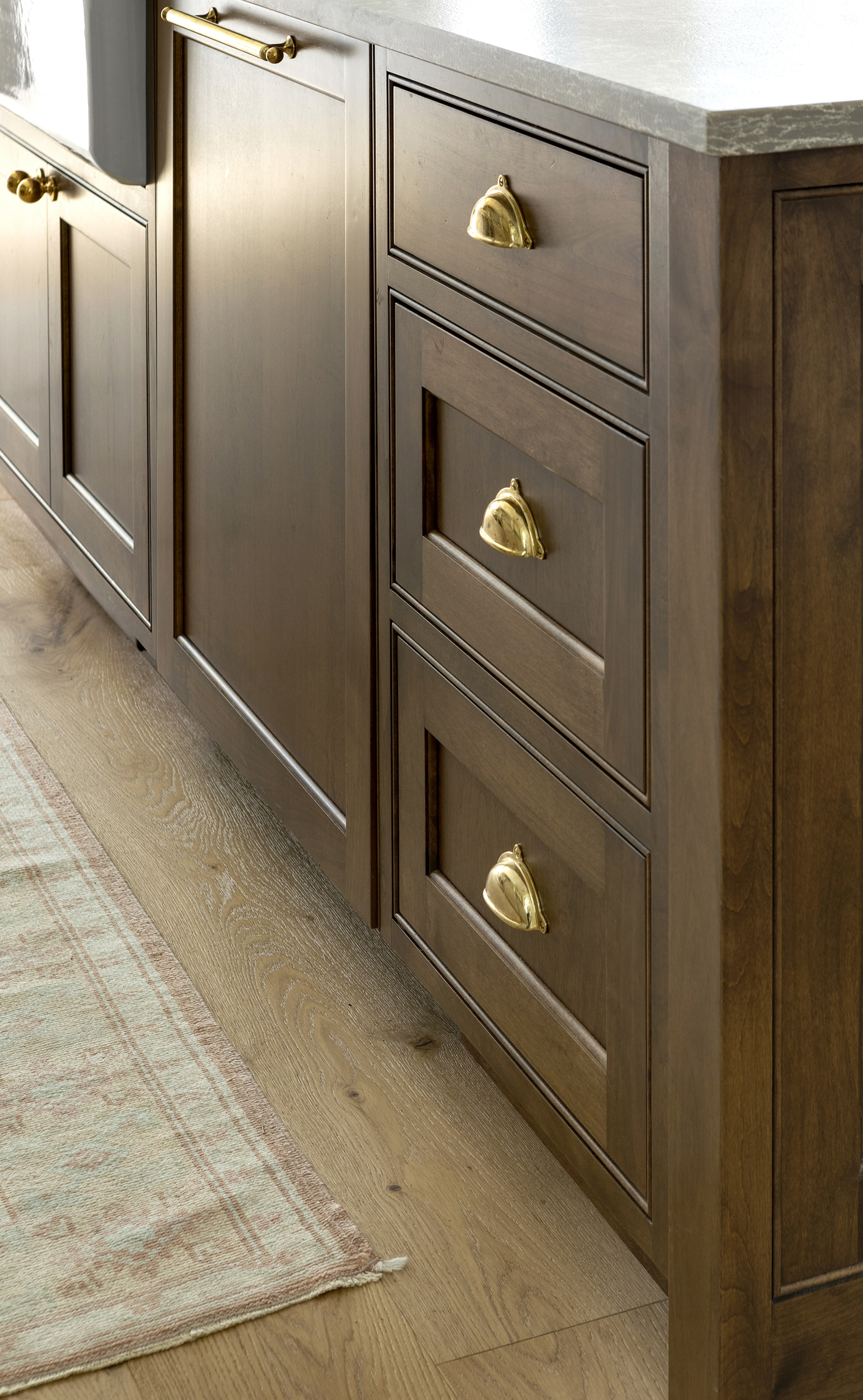This indoor color photograph captures a detailed view of a traditional-style kitchen corner. The focus is on a set of dark brown hardwood cabinets, potentially mahogany, adorned with eye-catching golden brass shell-shaped handles. The scene reveals a three-quarter side profile of the cabinetry, showcasing three vertically aligned drawers. The cabinets are topped with a sleek gray quartz countertop. In the upper left corner of the image, part of a white porcelain sink is visible, set against the same quartz surface.

The kitchen's flooring consists of unfinished light tan wooden floorboards, adding to the rustic farmhouse aesthetic. Laid across the floor is a thin, well-worn rug that adds a sense of homey charm. The room is well-lit, emphasizing the clean, new appearance of the cabinets, which show no signs of wear or tear. This photograph evokes the warmth and tradition of a classic kitchen setup.